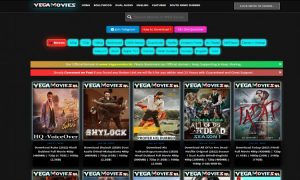The image depicts the Vega Movies website, which showcases various movies available for viewing or download. At the top of the webpage, there is a header labeled "Vega Movies," accompanied by a navigation bar with links to sections such as Home, Movies, Dual Audio, Web Series, and various genres. Below this navigation bar, there are several distinct colored tags likely representing different movie categories, such as New Hollywood, Bollywood, South Indian films, and web series.

The movie listings feature titles such as "HQ Vendor Box," "Shylock," "Movie 3," "All of Us Are Dead," and "Tezak." The website design utilizes a dark background complemented by bright colors for visual appeal. However, the overall look of the site suggests it may be a dubious subscription service, enticing users with promises of extensive movie libraries. The site's offerings appear questionable, potentially consisting of low-quality or obscure films, possibly filmed with amateur equipment. The service seemingly targets unsuspecting users by offering a subscription model that might not deliver on its promises.